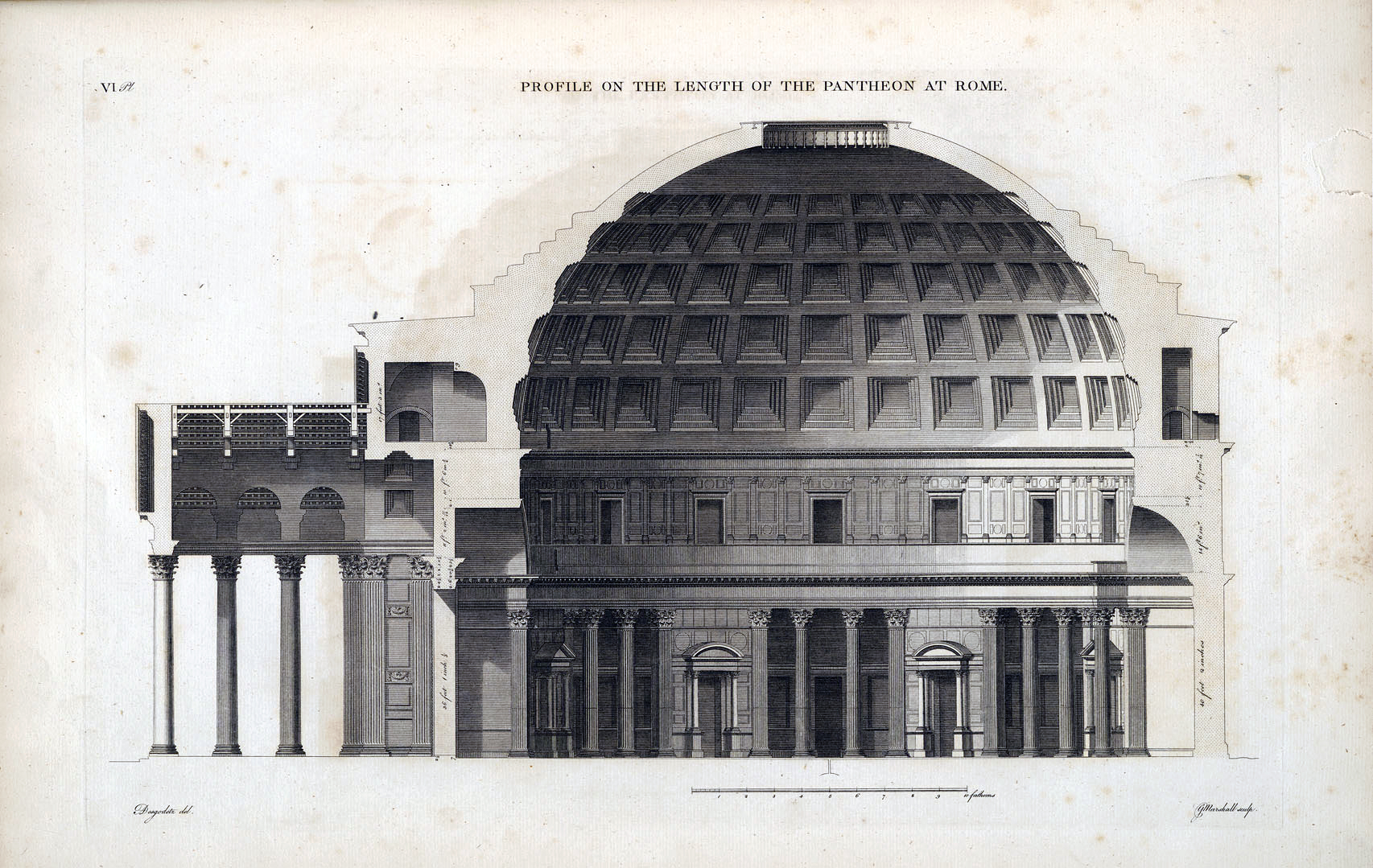The image is an aged, black-and-white architectural drawing, featuring the profile of the Pantheon at Rome. The drawing is done on yellowing, browning paper with worn-out patches, which adds to its antique look. Across the top, the text reads "Profile on the Lenoth of the Pantheon at Rome." The depicted structure is predominantly circular, capped with a large, segmented dome comprising layers of square sections that grow smaller towards the top. Below the dome, there are twelve layers of square segments that decrease in size as they ascend, with a small, plain section at the very top. The upper level of the building features numerous doorways lined along the floor, while the lower level showcases slender, fluted columns interspersed with additional doorways. On the left side, there is a wing supported by smooth, extra-long columns, leading to what appears to be an arched balcony. Smaller, barely readable text is scattered throughout the drawing, labeling various parts of the structure.